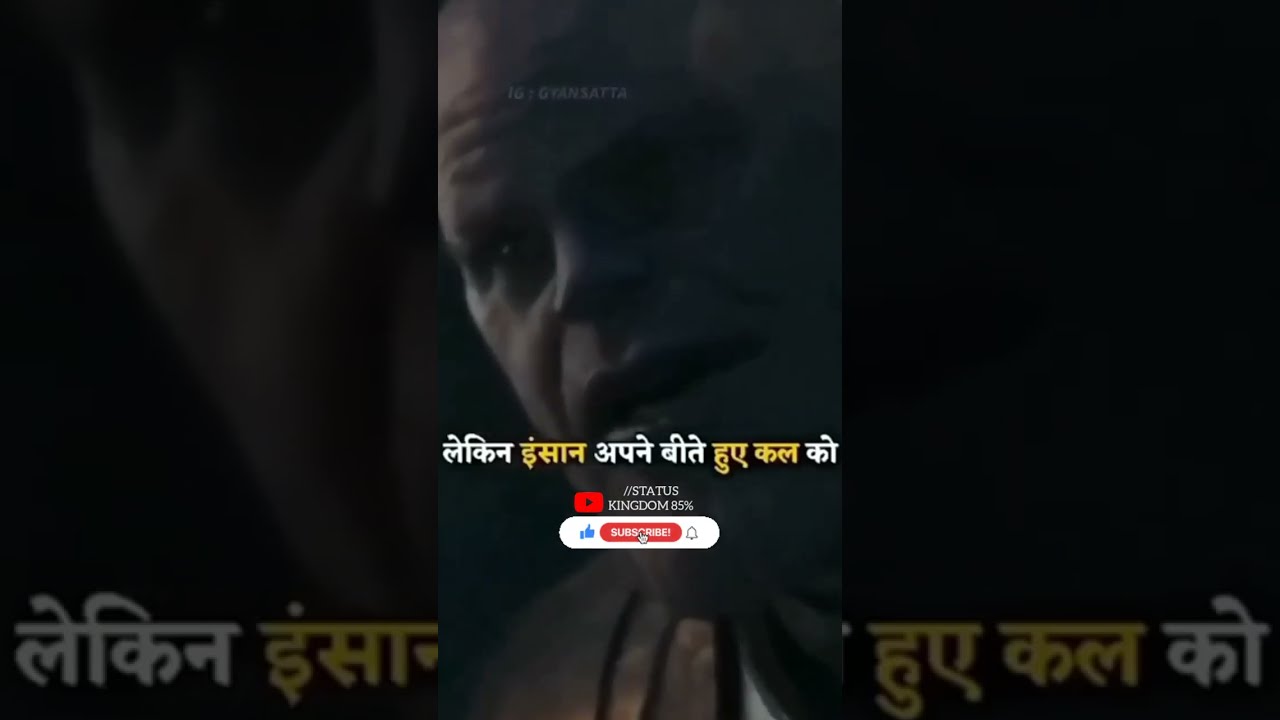The image is a dark, out-of-focus screenshot featuring a humanoid creature centered in the frame, showing a wrinkled forehead, deep-set eyes, and a partially opened mouth revealing some teeth. This creature appears to be wearing a brown, pleated material. The image includes foreign writing, possibly Arabic or Indian, both at the center and bottom of the picture. At the bottom, it reads "Status, Kingdom, 85%" followed by icons for a thumbs up, a bell, and a red "Subscribe" button. The left and right borders of the image are wide and contain heavily tinted and magnified sections of the central face, highlighting portions such as a corner of the chin and cheek, with the foreign script also magnified in these borders. The overall palette is predominantly dark, featuring black with white and yellow text, creating a mysterious and somewhat ominous effect.